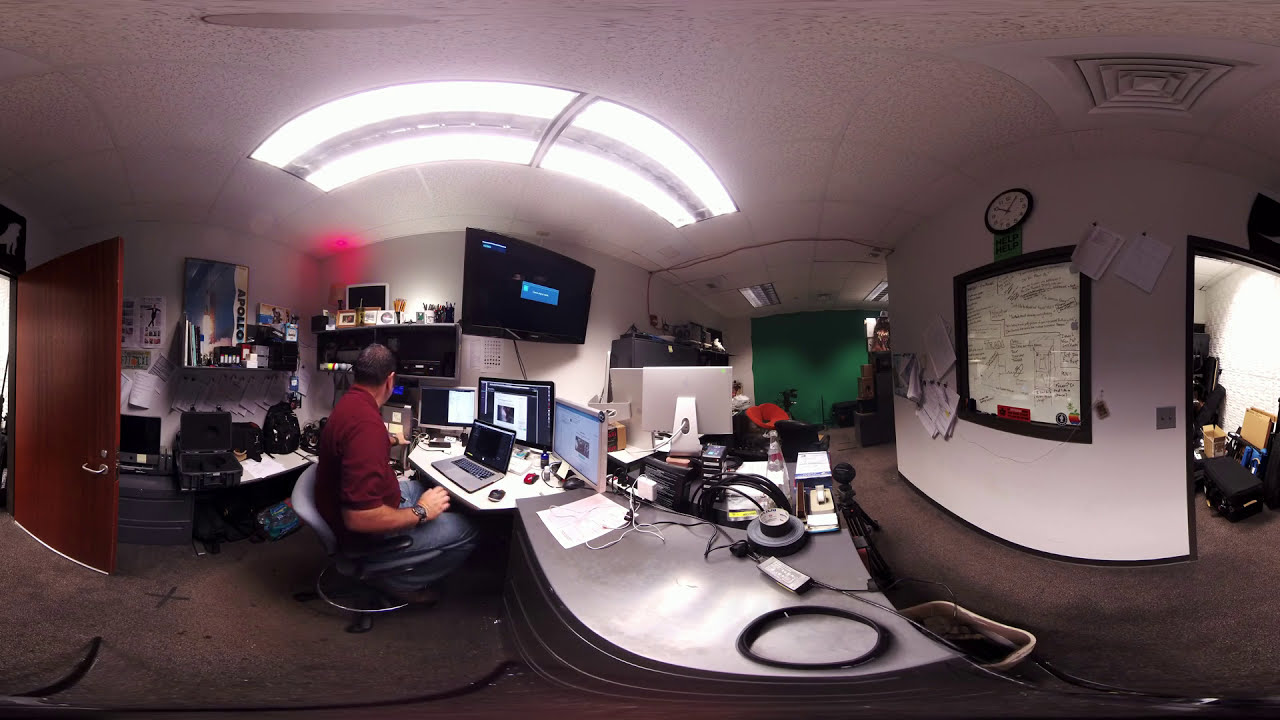In the image, we observe a man with brown hair, donned in a burgundy polo shirt and blue jeans, sitting directly in the center of a spacious office. He is stationed at a long, somewhat cluttered desk, featuring a laptop and multiple monitors with various electronic equipment scattered around. The man is wearing a black watch on his right hand. The office, set on brown carpeting, appears to function as a workshop given the plethora of computers, electrical components, and other technological devices.

Directly behind the man, shelves, racks, and drawers brim with equipment, including books and a backpack. Above him, a TV that seems newly turned on is mounted on the wall amidst other décor, such as posters and images, including one of the Apollo space capsule. 

To the left, there's a doorway leading to another room. To the right, a window with an attached whiteboard is visible, covered in numerous papers. Another doorway on this side opens into what looks like a storage room. Additionally, in the background on the right, there is a clock on the wall and a green-painted wall, with another person possibly seen further back. The office space is illuminated by both a pink light and a ceiling light, amplifying the array of colors in the scene, including tones of gray, white, purple, pink, red, green, black, and blue, contributing to the detailed and dynamic workspace atmosphere.